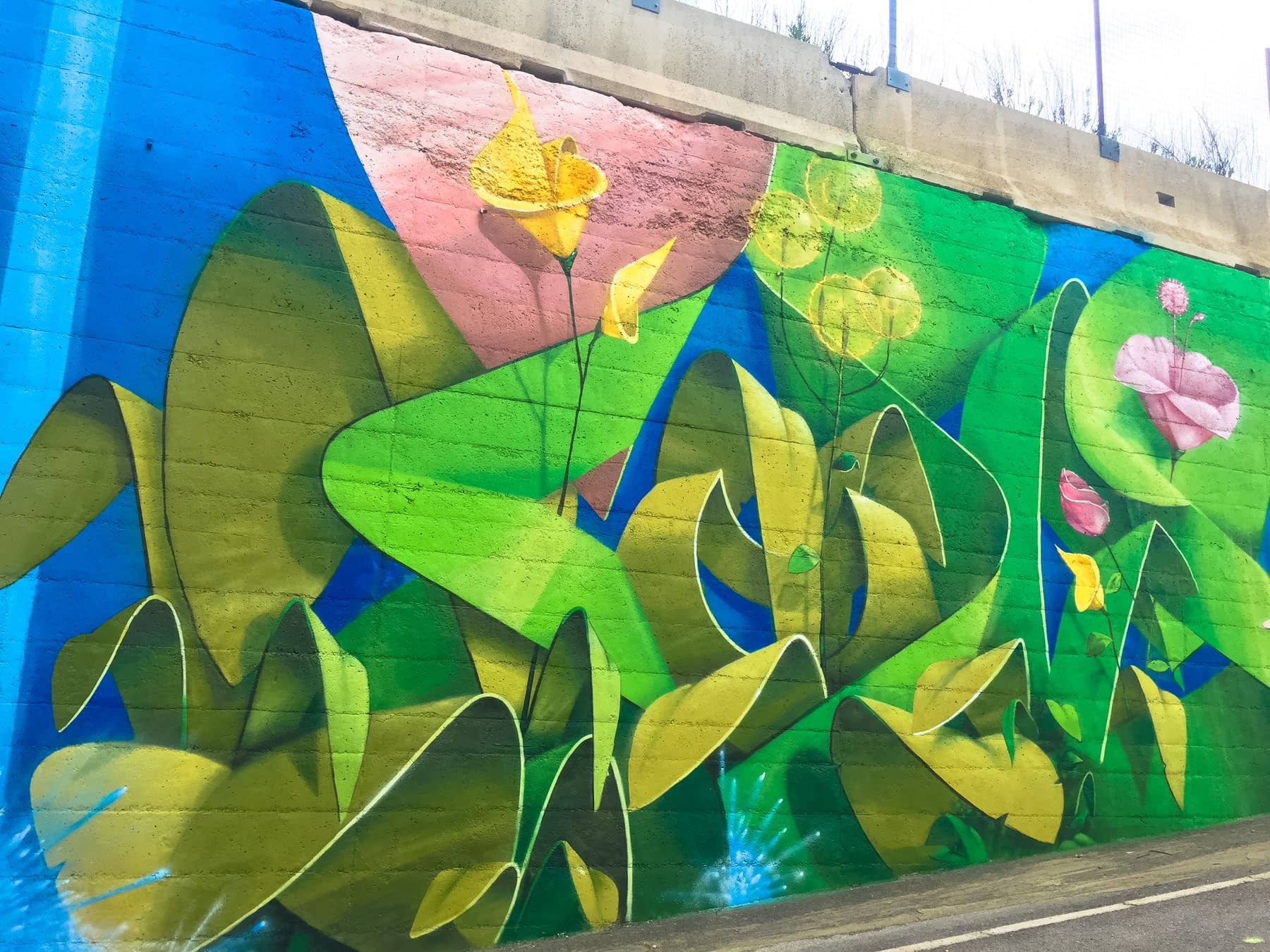This daytime image captures a vibrant outdoor scene featuring a large concrete wall, possibly a tunnel or berm, adorned with intricate spray-painted artwork. The wall showcases a stunning floral design, rich in various colors such as blue, green, dark green, yellow, pink, and light blue. The floral mural includes detailed tulips, roses, and other flowers, with leaves bending and framing the artwork on both the left and right sides. A road or path runs along the bottom of the image, with some grass and plants visible at the top, blending nature with urban art. The sky is overcast, adding a white backdrop above the fence and plant life growing along the upper part of the wall.